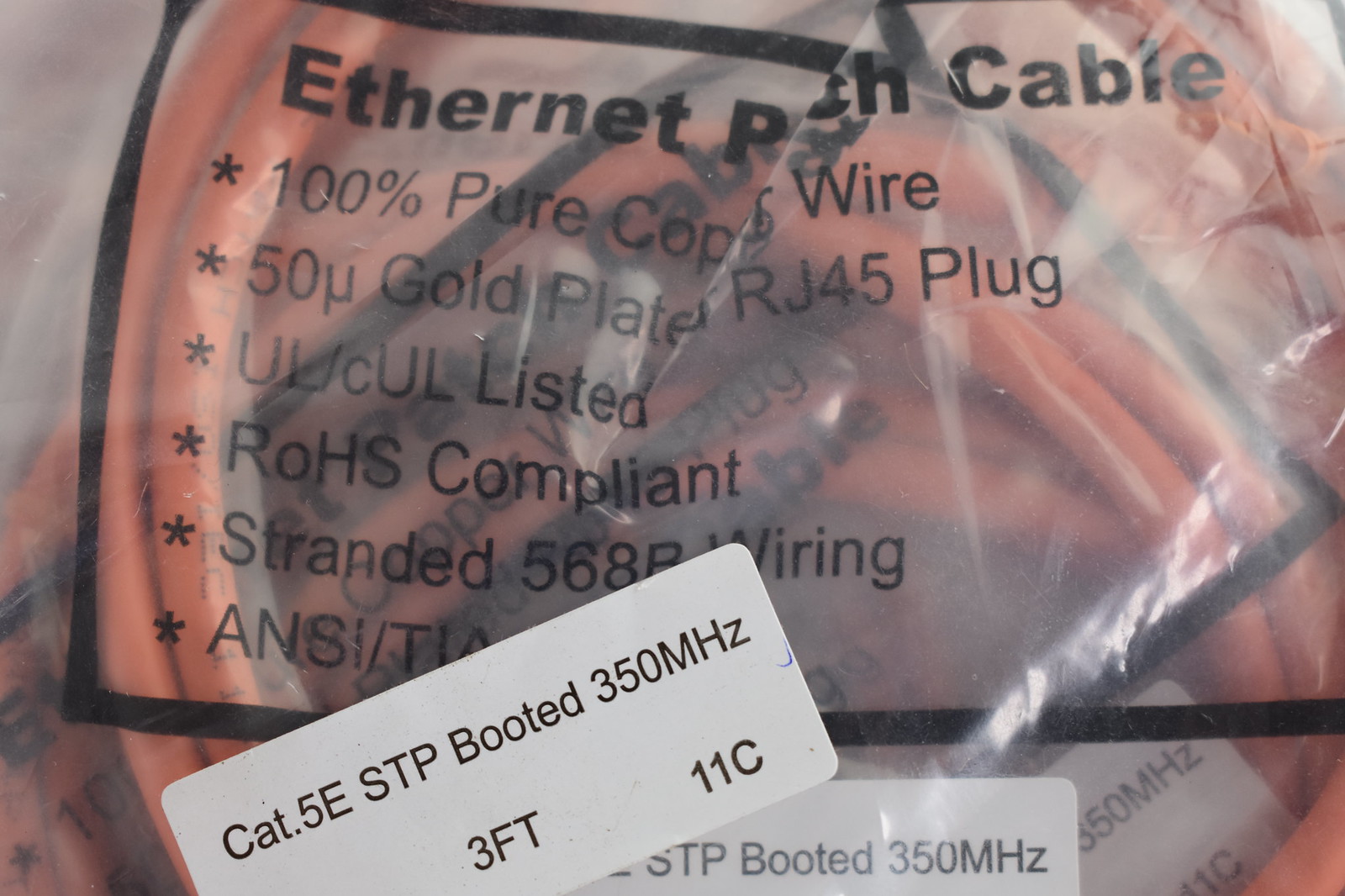The photograph, captured in landscape view, depicts an Ethernet cable still in its clear packaging. The visible orange cable is housed in a slightly wrinkled plastic bag. The bag features black printed text, partially obscured due to the folds. The print appears to have a black border, and the legible portions read "Ethernet" with an indistinct term following it, and "cable" underneath. Below this heading, there are three bullet points listing: "100% pure copper wire," "50U gold plate RJ45 plug," "UL, CUL listed," "ROHS compliant," "stranded 568P wiring," and "ANSI-T..."—which is partially obscured by a sticker. This white sticker, with black text, reads "Cat. 5E STP booted 350 MHz 3 feet 11C." Another sticker, located at the bottom, similarly states "Cat5E booted 350 MHz." The clear packaging allows for the orange wiring inside to be distinctly visible.